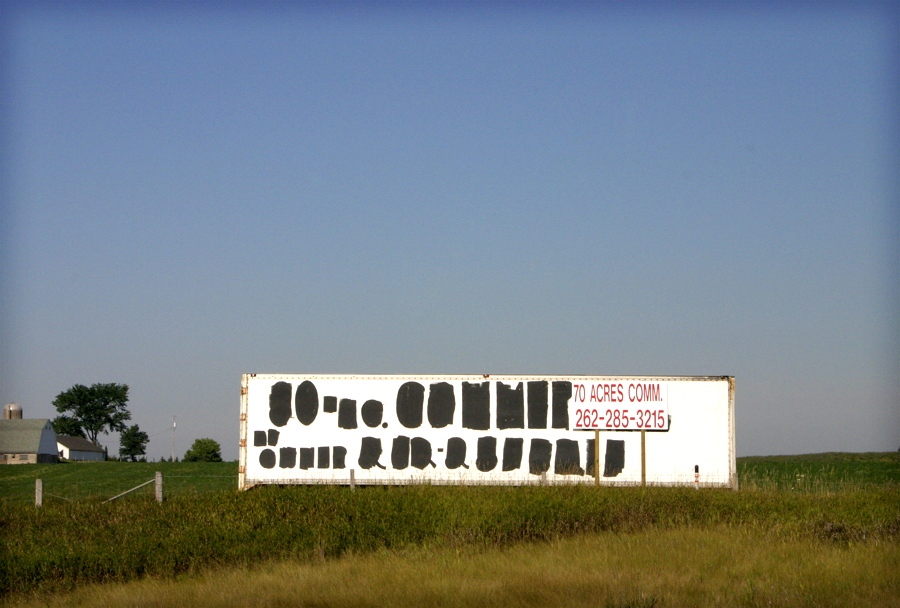This photograph, taken outdoors on a clear day, captures an expansive rural scene dominated by an empty, wide billboard. The bottom of the image reveals a stretch of brown grass, suggesting a parched or non-irrigated area, transitioning into lush green fields in the background. To the left of the billboard, a quaint farmhouse and barn are nestled among a few trees, enhancing the rustic charm of the setting. The sky starts off as a pale blue near the horizon, gradually darkening to a richer blue higher up, dotted with sporadic clouds. The billboard itself is prominent, occupying about half of the frame horizontally and is perfectly centered across the width of the photograph but positioned below the vertical midpoint. The white surface of the billboard is marred by irregular black marks, likely from torn material or haphazard paint. In the foreground, a smaller sign reading "70acrescomm" followed by a phone number, "262-285-3215," stands as a stark contrast against the expansive rural backdrop.